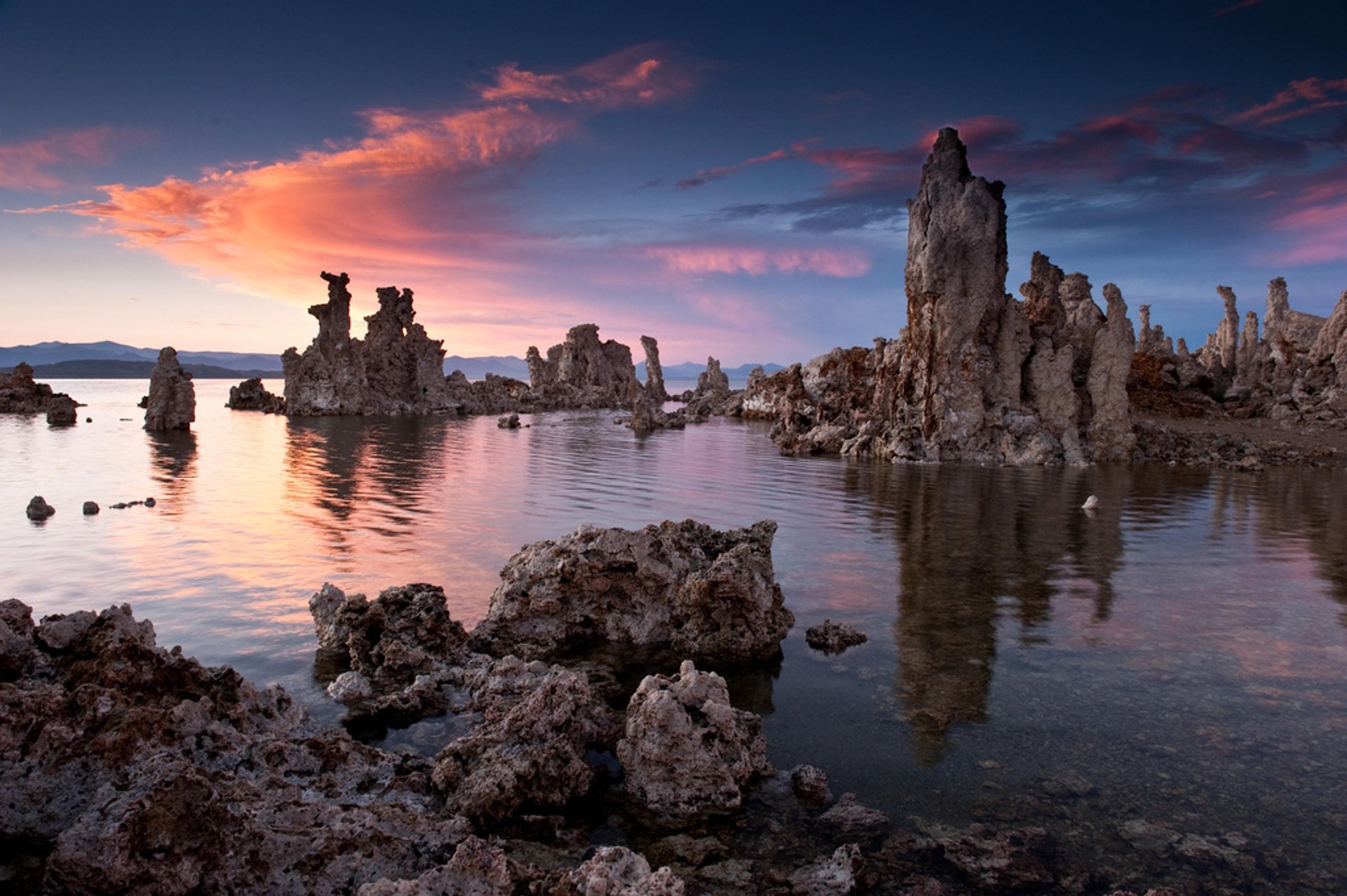A mesmerizing seascape unfolds under a vivid, deep blue sky, adorned with a striking pinkish-orange cloud shaped like a bird gliding towards the left. The scene is framed by a menacing array of jagged rocks, likely volcanic, that juts menacingly from the sea. These sharp formations rise like pillars, forming an intimidating and unyielding reef that would easily breach the hull of any ill-fated ship that approached too closely. In the distance, beyond the perilous rocks and the expansive, open waters, the tranquil outline of land is visible, contrasting sharply with the foreboding foreground. The overall impression is one of awe at nature's beauty mingled with a deep sense of caution.